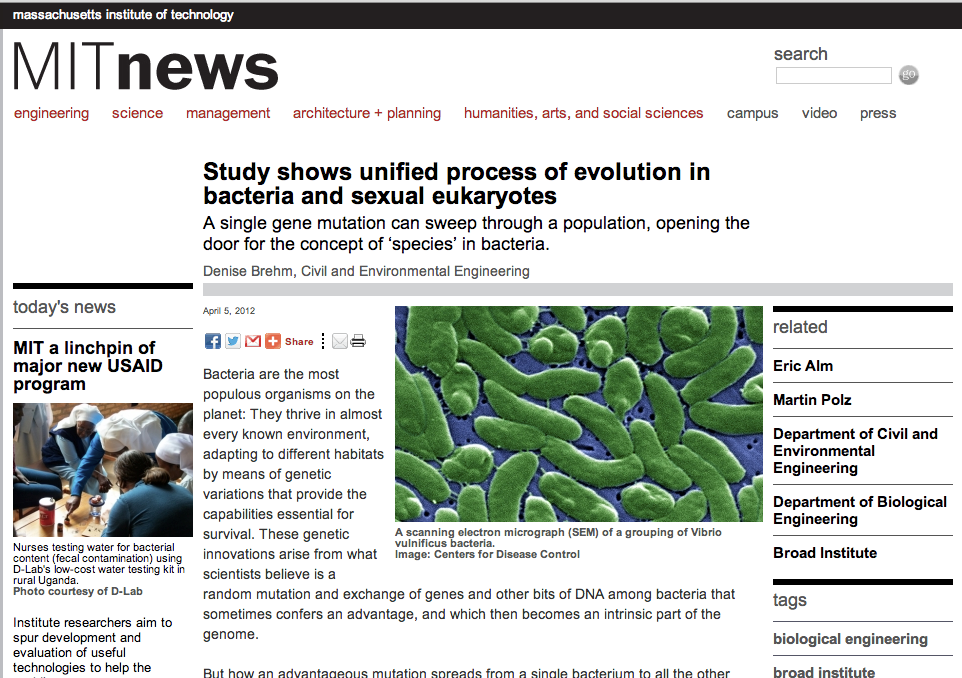This is a detailed screenshot of a web page from the Massachusetts Institute of Technology (MIT). The top of the page prominently features "MIT News" in black. There are several navigational buttons available for users to filter content, including categories like Engineering, Science, Management, Architecture + Planning, Humanities, Arts, and Social Sciences. Additionally, there are buttons labeled Campus, Video, and Press, with the majority of the buttons displayed in red, and the last three in gray.

The featured news topic on this page is "Study Shows Unified Process of Evolution in Bacteria and Sexual Eukaryotes," accompanied by a close-up microscope image depicting green bacteria. To the far left, there is another news article titled "MIT, a Linchpin of Major New USAID Program." This article includes an image showing a group of people, mostly dressed in blue with white hats, who are described as nurses testing water for bacterial content. On the right-hand side of the page, there are sections labeled "Related" with references to individuals such as Eric Alm and Martin Polz, along with links to additional related information.